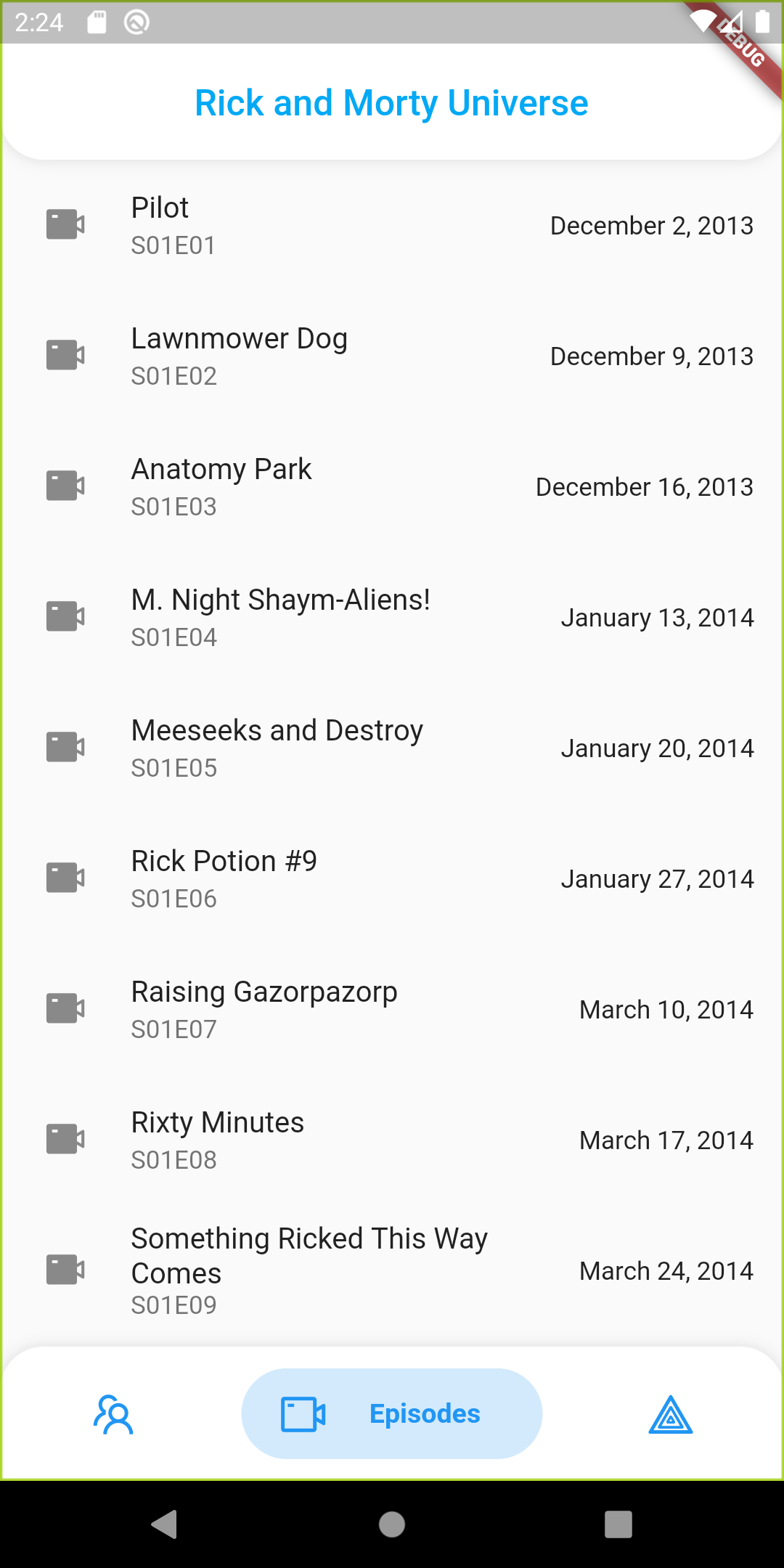This is a detailed screenshot of a smartphone screen in a vertical orientation. The top of the screen displays the time "2:24" in white on a light gray banner, which also contains typical status icons in white, including a battery indicator and signal strength. In the top right corner, an additional icon, a sideways triangle, is present. Cutting across the top right corner is a red banner with "DEBUG" written in white letters.

Just below this, centered at the top on a white background, is the text "Rick and Morty Universe" written in a light royal blue color. Below this title, the screen displays a list of clickable items resembling video thumbnails, most likely episodes from the show. Each episode listing includes a small light gray video camera icon next to the episode title, with the first episode titled "Pilot" in black text. Accompanying details include the episode number "S01E01" and the release date, "December 2nd, 2013."

The listing continues down the page, showing a chronological progression of episode titles and dates, such as "Something Ricked This Way Comes," dated "March 24th, 2014." Toward the bottom of the screen are additional images of people, episode titles, and more clickable icons, including a triangle symbol.

This detailed screenshot provides a comprehensive view of a phone screen displaying "Rick and Morty" episodes, complete with associated metadata and user interface elements.